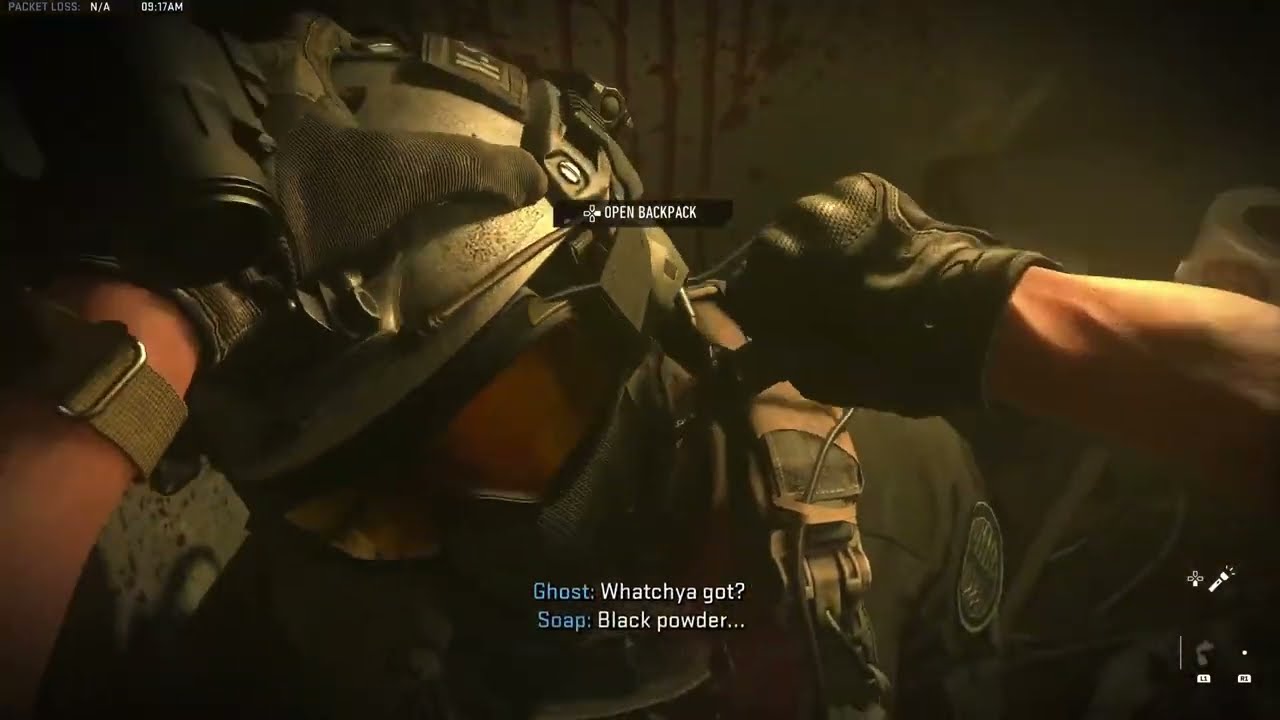The image depicts a detailed screenshot from a campaign mode of a video game, presenting a tense scene involving two soldiers. Dominating the foreground is a soldier in full combat gear, including a large, gray military helmet, black leather gloves, and a green camouflage uniform with visible backpack straps and an emblem on the left shoulder. His yellowish-orange goggles contrast against the peach tones of his skin. The soldier's left hand is gripping his helmet, while his right hand appears to be forcefully pressing into another character's neck, with a hint of red blood suggesting a stabbing motion.

The background features a greenish-brown hue that adds to the intense atmosphere. Overlaying the image are various game interface elements. In the top left corner, there is an icon indicating "packet lost, not available." Centrally positioned text reads "open backpack," accompanied by a keypad icon with the right section highlighted. In the lower right corner, another keypad icon has the lower key highlighted next to a flashlight icon.

At the bottom, enclosed captions display a conversation in blue text: "Ghost: What you got" to which "Soap" responds, "Black powder," both in white text. The gripping visual combined with the interactive prompts and dialogue suggest a critical moment in the gameplay narrative.